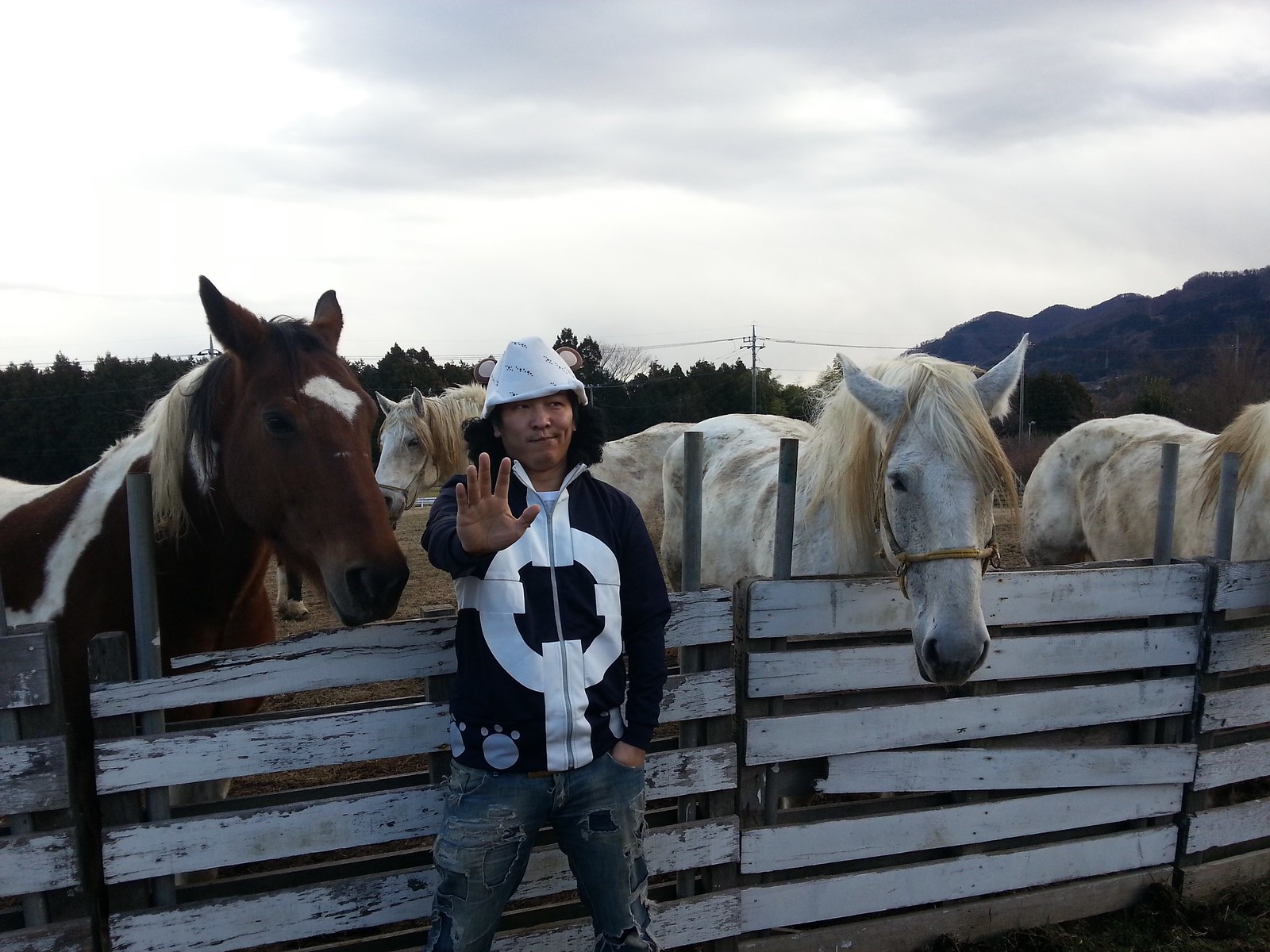This outdoor photograph captures a man standing in front of a weathered white wooden fence, partially stripped of paint. Behind him are four horses—three of them are white with flowing white manes, and the one on the left is brown with distinctive white spots, including a diamond-shaped patch on its forehead. The man is dressed in heavily patched blue jeans and a dark blue zip-up jacket with white decorative elements. He wears a unique white hat adorned with dark decorations. His right hand is raised in a gesture resembling a stop signal, palm outstretched and fingers pointing upwards, while his left hand rests in his pocket. He has a slight, amused smirk on his face and is looking amusedly off to the side of the camera. His stance is relaxed, with legs slightly apart. The backdrop features trees, a small mountain or hill, and visible electrical or telephone wires, all under a cloudy sky, indicating it’s a daytime shot. The scene captures both the rustic charm of the fence and the natural beauty of the horses and surrounding landscape.